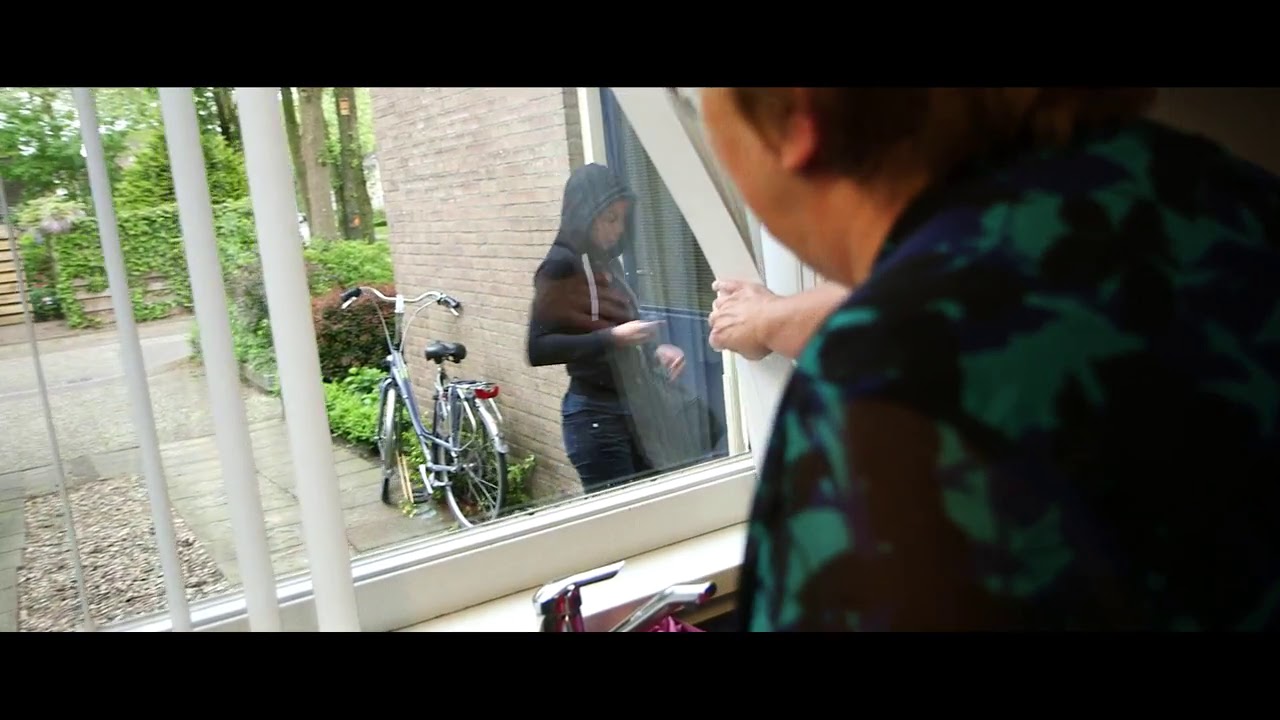The photograph, framed with a black bar at the top and bottom reminiscent of a theatrical or cinematic presentation, features an older woman with brown hair and fair skin, wearing a green and blue floral shirt. She is pulling back white blinds over a kitchen window with a visible faucet, suggesting it's positioned above the sink. Her expression appears concerned or suspicious as she gazes out.

From the woman's vantage point, a young woman in her early 20s is seen standing in front of a blue door at the corner of the house, extracting a key from her bag or possibly holding a phone. The young woman is dressed in a black hooded sweatshirt and black pants, with a bag slung over her shoulder. The house, made of pale bricks, has a brick walkway leading to the door. To the left of the door, a dark blue vintage bicycle with silver trim leans against the wall. Beyond the house, the scene includes lush greenery, such as trees, ferns, and other plants, enhancing the overall natural ambiance. The detailed composition and the observer’s stance through the window suggest a moment of tension or curiosity.